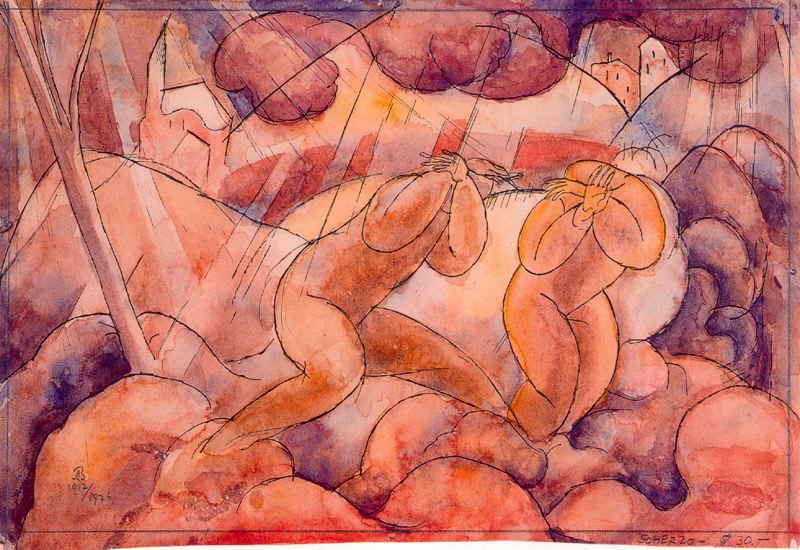This image is an abstract watercolor painting characterized by vibrant shades of peach, red, orange, and purple, accentuated with a thin black line pencil sketch. Dominated by caucasian peach-pink flesh tones, the artwork presents a surreal and interpretive scene. At its center are two naked, genderless humanoid figures with their arms raised, obscuring their faces. The figures are depicted with rounded heads, universal torsos, arms, hands, fingers, and legs, but without feet, breasts, or genitalia. Surrounding them are amorphous shapes and blobs, which evoke a sense of body fat or blubber, some of which seem like clouds or rocks. The background includes a tree to the left, and distant structures that resemble buildings, or perhaps a church. The composition suggests a haunting atmosphere with a spectrum of warm colors, numerous undulating forms, and an overall sense of ambiguity and complexity.